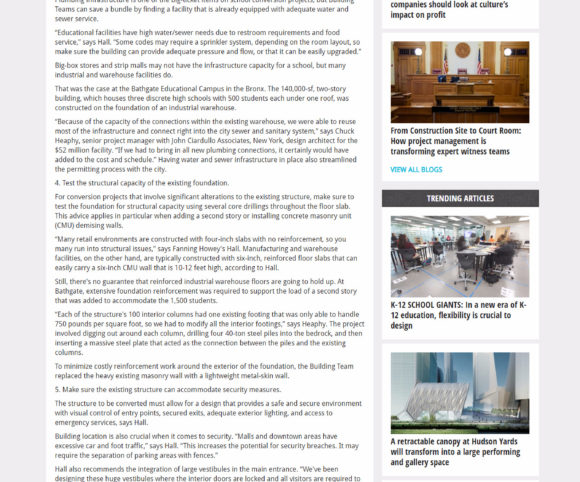The image is a screenshot of an article viewed on a mobile device or computer. The article is displayed on a white background with black text, bordered by gray margins on either side. The content is interrupted by three photographs aligned to the right. One photo depicts a formal courtroom, complete with American flags, a circular crest, a raised wooden desk, and two ornate white globe lights. The wood paneling and accents are prominent within the courtroom. The accompanying text above the photo reads: "From Construction Site to Courtroom: How Project Management is Transforming Expert Witness Teams." Below the photo, there is a blue hyperlink titled "View All Blogs."

Additionally, there is a section titled "Trending Articles," highlighted by a black banner. One of the trending articles is titled "K through 12: School Giants in a New Era of K-12 Education," discussing the importance of flexibility in school design. This section is visually supported by an image of a brightly lit classroom.